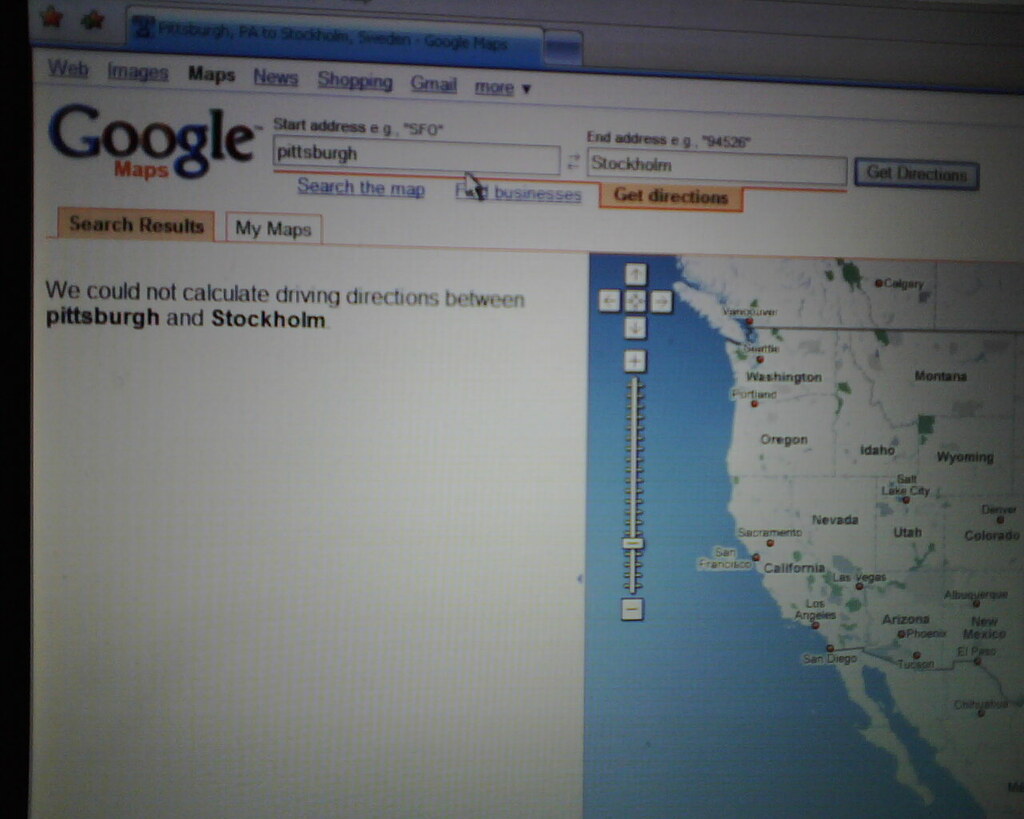A vintage computer monitor displaying a dated web browser—reminiscent of late Internet Explorer versions—shows a Google Maps results page. Despite the aged interface, the Google UI appears relatively recent. The search on the screen seeks driving directions from Pittsburgh to Stockholm, Sweden. The Maps tab is active, and the left panel states: "We could not calculate driving directions between Pittsburgh and Stockholm." This message confirms Google’s interpretation of 'Stockholm' as Stockholm, Sweden.